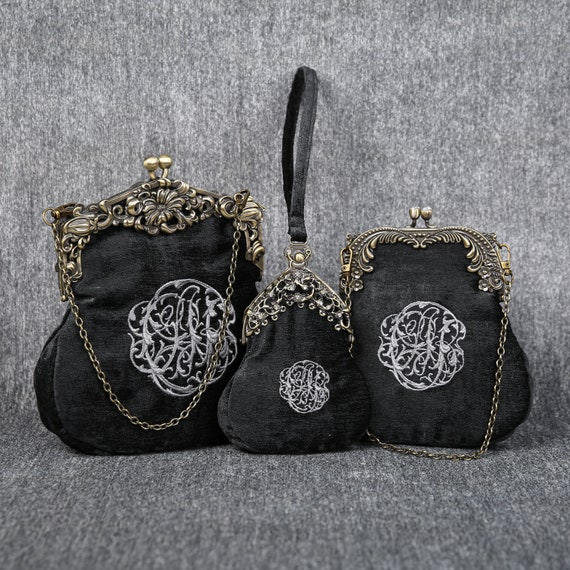Three exquisite black purses are elegantly arranged on a heather gray photographer's backdrop, which seamlessly drapes from the wall onto the floor. These nearly identical handbags vary in size, with the largest positioned on the far left, the medium-sized one on the far right, and the smallest centered between them.

Each purse features intricate, silvery-white embroidery forming ornate circular designs on their surfaces, reminiscent of delicate lacework vines. The bags are adorned with ornately worked metal tops, adding a touch of sophistication to their look. 

The largest and the medium-sized handbags are equipped with short metal chain handles, suitable for holding in one hand. Meanwhile, the smallest bag, positioned in the center, stands out with a flat black wrist strap secured by a sturdy metal attachment. The collective design elements emphasize both elegance and functionality, making these purses a striking visual ensemble against the neutral backdrop.